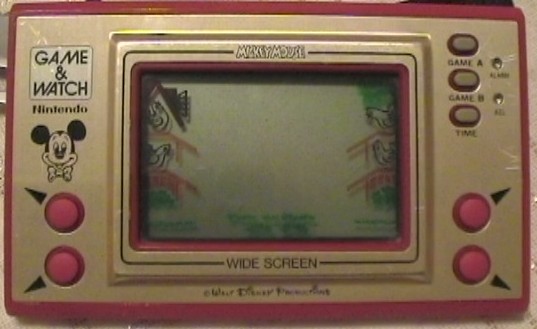This photo features an old-school handheld Nintendo gaming device with a gold-pink body, accented by a red rectangular border. The screen, labeled "widescreen" below, is situated in the center with minimal green and black coloring, indicating an inactive state where typically it would light up in black and white. The device is distinctly themed with a Mickey Mouse motif, carrying a logo and label of "Walt Disney Productions" underneath the screen. On the left, it states "Game & Watch Nintendo." There are two red buttons on both the lower left and lower right sides, each marked with black arrows pointing outward. The buttons on the right are labeled "Game A", "Game B", and "Time." This gaming device, endorsed by familiar Disney imagery, was a popular single-game console from childhood eras past.